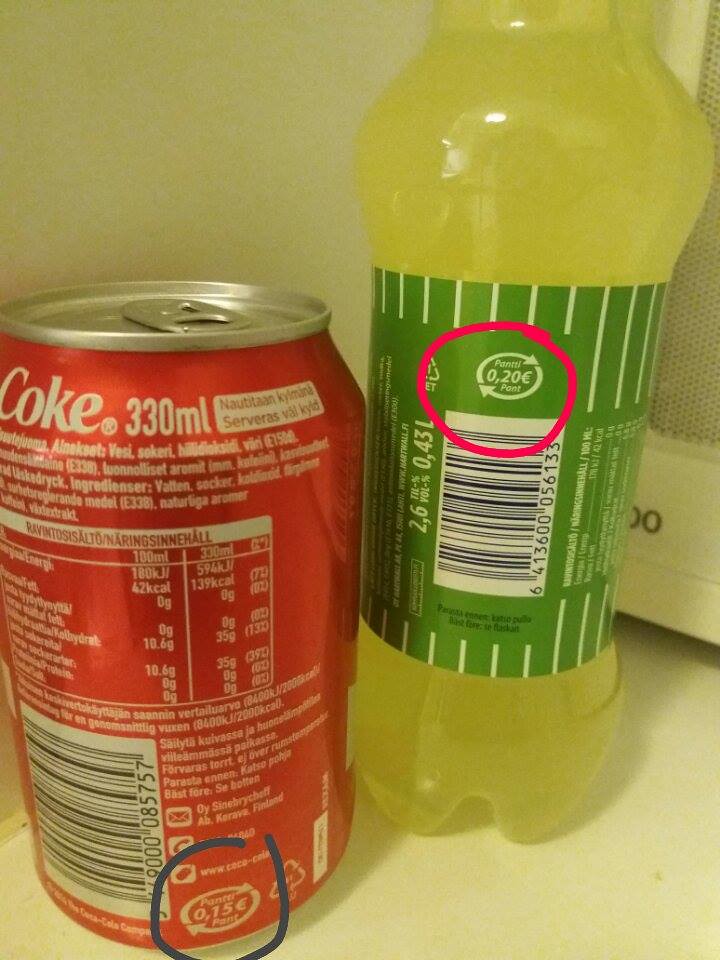A detailed image caption could be:

"In this image, there is a red Coca-Cola bottle positioned on a white tabletop, rather than inside a refrigerator. The focus is on the back of the bottle, which features a partially circled marking in black marker near the bottom that highlights something with a 'P' and '15'. The Coke bottle displays typical nutritional content information and volume measurements in milliliters, along with a UPC bar code. Adjacent to the Coca-Cola bottle is a green bottle with a green label, which is similarly marked with a red circled annotation that reads '.2E'. Below these bottles lies a white object, possibly a device with a small screen similar to a microwave display, and the last visible characters on this object are '00'."